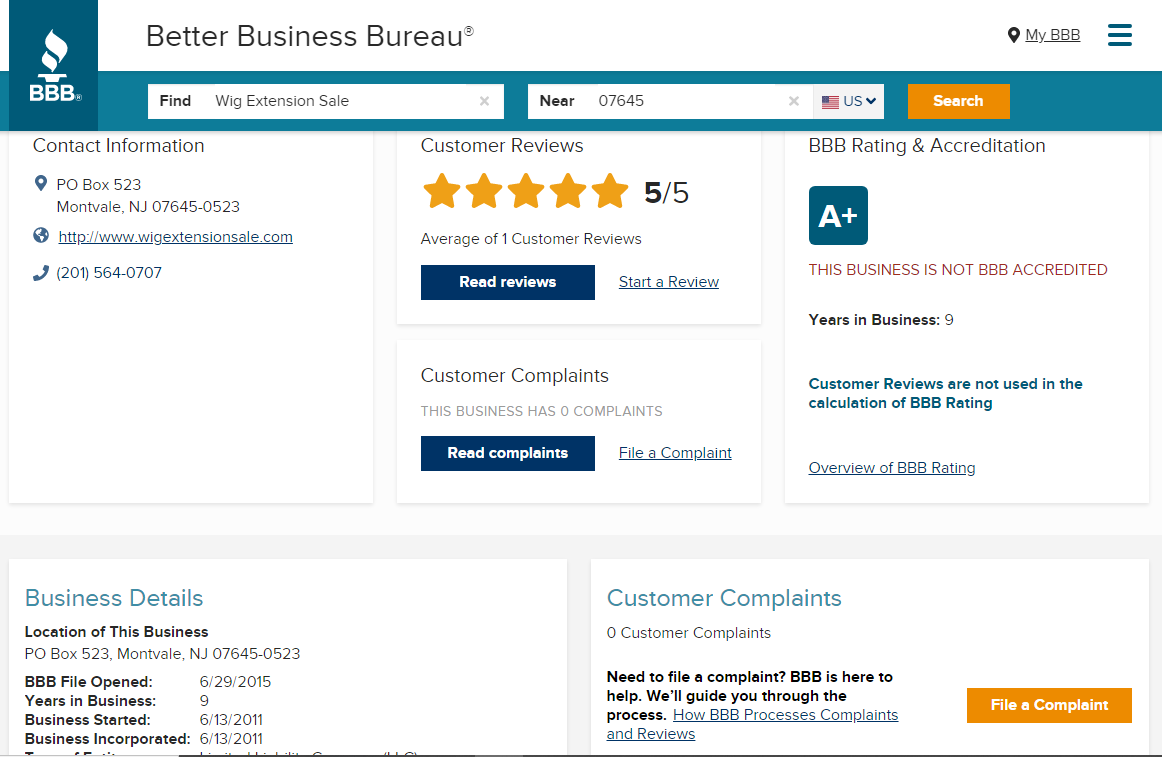This is a detailed and descriptive caption of an image showcasing a segment of the Better Business Bureau (BBB) website:

The screenshot captures the Better Business Bureau (BBB) website interface. At the top of the image, the BBB logo, comprising a white bar on the left with a dark blue rectangle featuring the BBB emblem and "Better Business Bureau" text, is prominently displayed. Directly below is a horizontal blue navigation bar containing a pair of search fields. The first field, labeled "Find," is a text entry box designed for inputting the name or type of business. Adjacent to it, on the right, is another white text entry field labeled "Near," intended for entering a geographic location or zip code.

Beneath the search fields, a business example is presented. The business, "WigExtensionSale.com," displays its contact information, including a phone number and address. Further details reveal the business's customer rating of five out of five stars, although this rating is based on a singular review. At the bottom of the description, a section titled "Business Details" is visible, followed by another labeled "Customer Complaints," indicating that this business has zero recorded customer complaints.